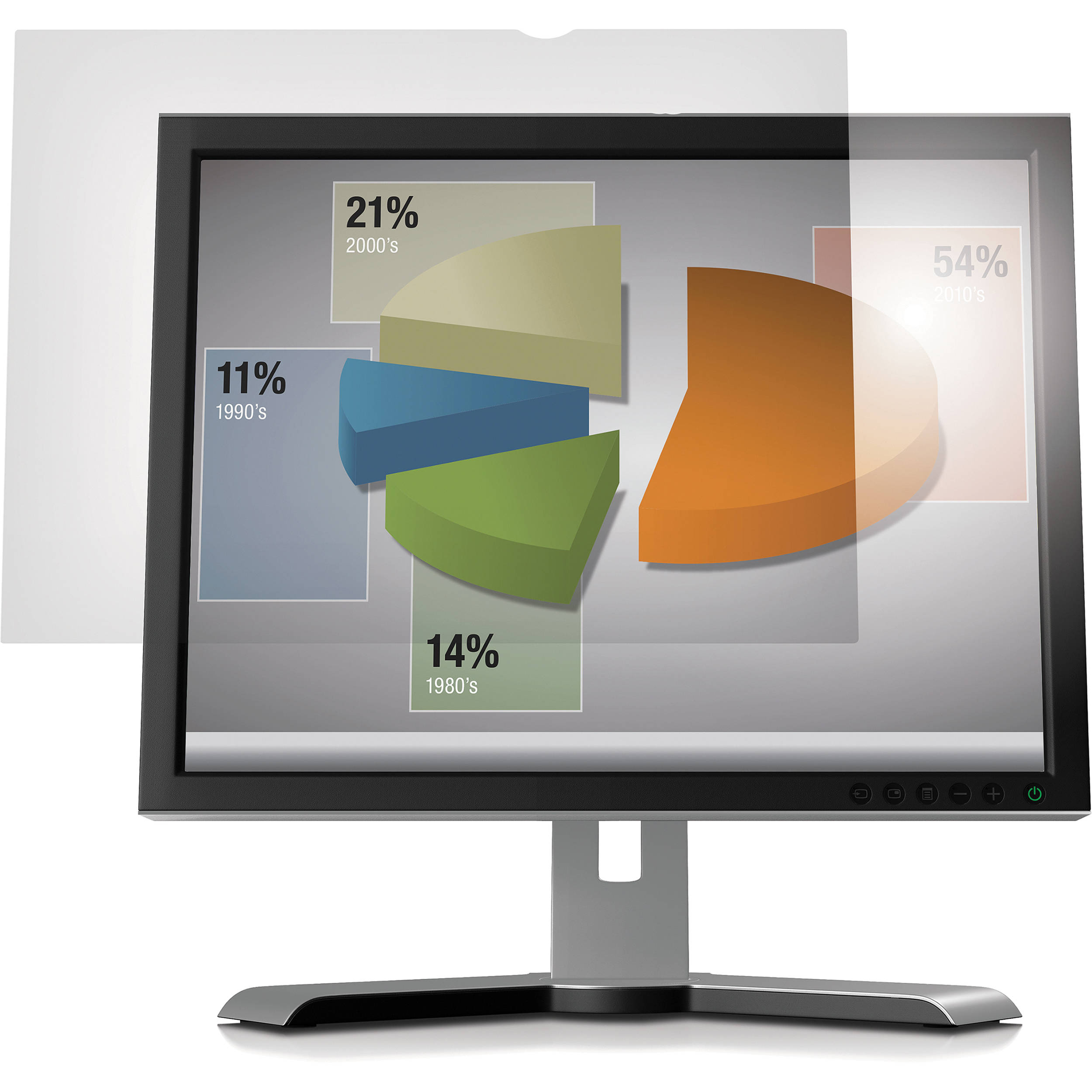This is a computer-generated illustration of a black monitor with a silver metal stand, featuring a circular graph or pie chart centrally displayed on the screen. The monitor stand includes a hole in the middle for cord management, and a green power button is located on the bottom right side. The pie chart is divided into four colored segments: an orange slice representing 54% for the 2010s, the largest segment occupying most of the right side of the chart; a yellow slice at the top representing 21% for the 2000s; a green slice representing 14% for the 1980s, the second smallest; and a blue slice representing 11% for the 1990s, the smallest segment. Additionally, there are faded, mirrored or "ghost" images of the monitor floating to the upper left, giving the impression of a superimposed or duplicate screen in the background. The colors used in the chart include orange, green, blue, yellow, beige, gray, and black. This detailed composition shows the percentages and corresponding years, organized consistently across the display.